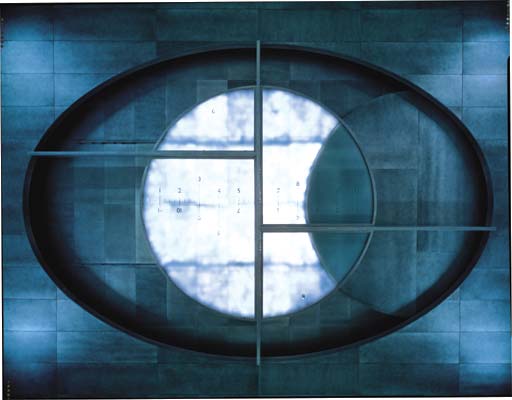The image is a highly detailed graphic or potentially a hyper-realistic painting, predominantly showcasing abstract shapes and intricate design elements. The overall composition is mostly square in shape, featuring a tightly packed backdrop of rectangular cinder blocks which are longer in width than height, and are uniformly colored in blue with darkened corners almost to black.

Central to this complex design is a large horizontal oval, resembling an eye or an egg, forming a ring of black. Running vertically down the center of this oval is a thin blue beam or pipe, with two additional blue pipes extending centrally outwards but in opposite directions—one towards the upper left and the other towards the lower right, stopping at the outer edge of the oval ring.

Inside this oval lies a perfect circle highlighted in subtle whites, giving it an illuminated appearance similar to a full moon or an eclipse. The circle is overlaid by a faint ruler marked with numbers 1 through 6 at the top and bottom, along with small vertical lines. Additionally, a partial circle in a regular blue tone overlaps the white circle on the right-hand side, enhancing the impression of a sliding door or disc-shaped region moving slightly to the right, exposing the left side while partially covering the right.

The blue and bluish-gray hues create a muted background, interspersed with bars resembling grates on a window, adding to the overall abstract and modernist aesthetic.